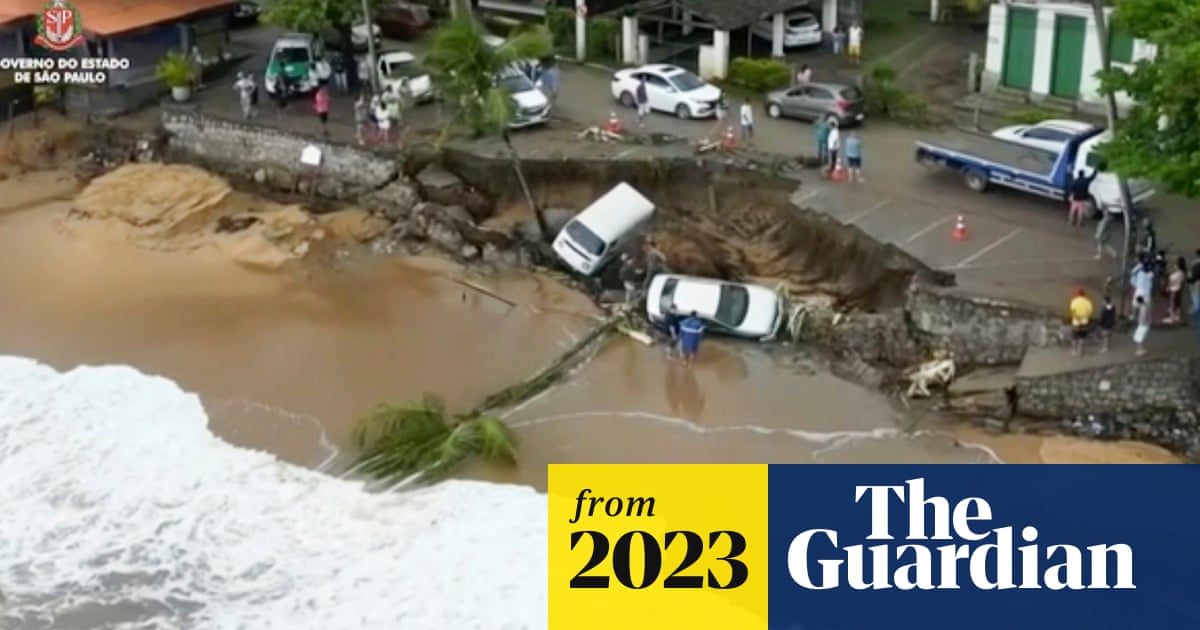The image, featured on The Guardian's website in 2023, depicts a dramatic scene of a natural disaster in São Paulo, Brazil. The setting is a collapsed road or possibly a parking lot adjacent to a beach, characterized by visible sand and sea waves rolling in. The collapse appears to be the result of a landslide or severe erosion, as evidenced by the fallen earth and debris. Two white vehicles have plunged into the sizable hole created by the collapse. The scene is crowded with onlookers and emergency responders, as evident by the presence of orange safety cones and a flatbed truck ready to retrieve the fallen cars. Among the fallen debris are two trees, including a palm tree, uprooted by the force of the collapse. The overcast, potentially rainy sky adds a somber tone to the image. In the background, several police cars with blue hoods are visible, as well as structures that look like buildings, including what might be a covered garage and other utility buildings, possibly bathrooms. This dramatic scene underscores the impact and aftermath of natural forces on urban landscapes.